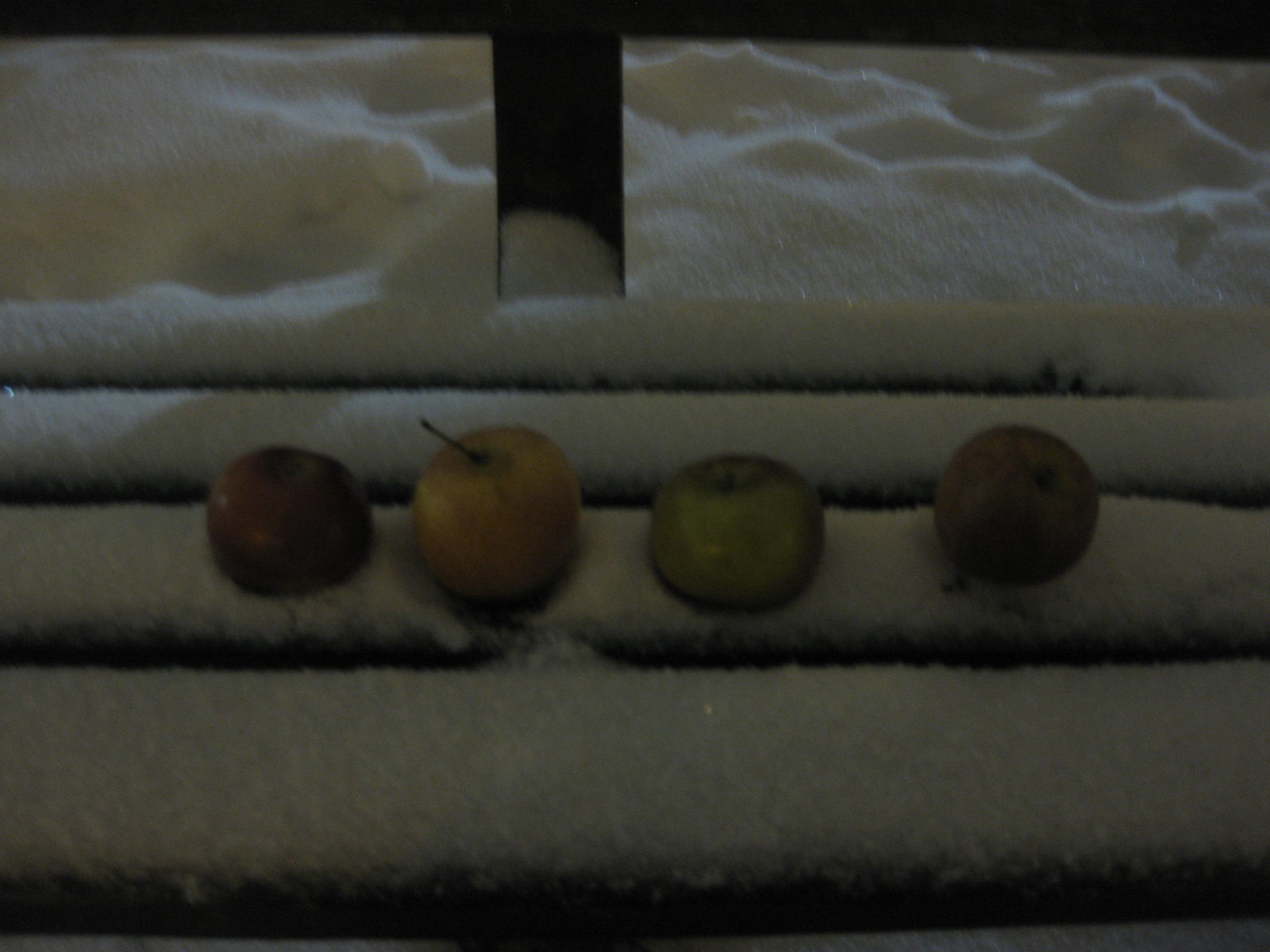This nighttime photograph captures a serene, snowy outdoor scene. Four apples are meticulously arranged on a snow-covered wooden surface, which could be steps or a bench. The photograph's darkness is subtly illuminated, possibly by moonlight, giving it a calm, ethereal glow. The background reveals a blanket of snow with wavy texture, suggesting recent accumulation.

In the forefront, wooden slats covered with several inches of snow horizontally traverse from left to right. On the second or third slot from the top, the apples appear equidistantly spaced. Starting from the left, the first apple is a vibrant red, the second is a reddish-yellow apple with a distinct stem, followed by a green apple, and finally, the fourth apple has a mixed red and green hue. Despite the snowy isolation, there are no visible footprints or any indication of human or animal presence, enhancing the sense of pristine solitude.